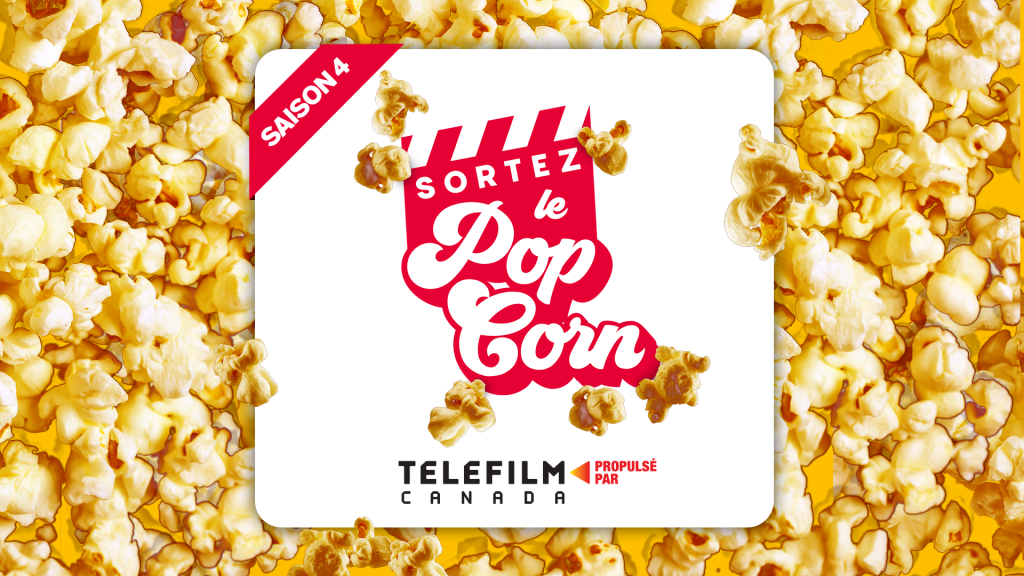This horizontal rectangular image appears to be a professionally made advertisement for popcorn, likely meant for display in a movie theater. The background is a flat sheet of yellow buttered popcorn, creating a vibrant and appetizing backdrop. Situated in the center of the image is a prominent white square. Across the upper left corner of this square is a red banner with the French text "Saison 4." In the middle of the white square, bold white letters on a red background spell out "Sortez le Popcorn." Below this, in black letters, are the words "Telefilm Canada." The white square is partially overlapped by popcorn kernels at its edges, adding a dynamic element to the design. Additionally, the image contains the text "Propulsé par" to the right, hinting at the advertisement's sponsorship. Overall, the use of red, white, and yellow colors makes the poster visually striking and effectively highlights the main elements, making it clear this is an alluring popcorn advertisement.